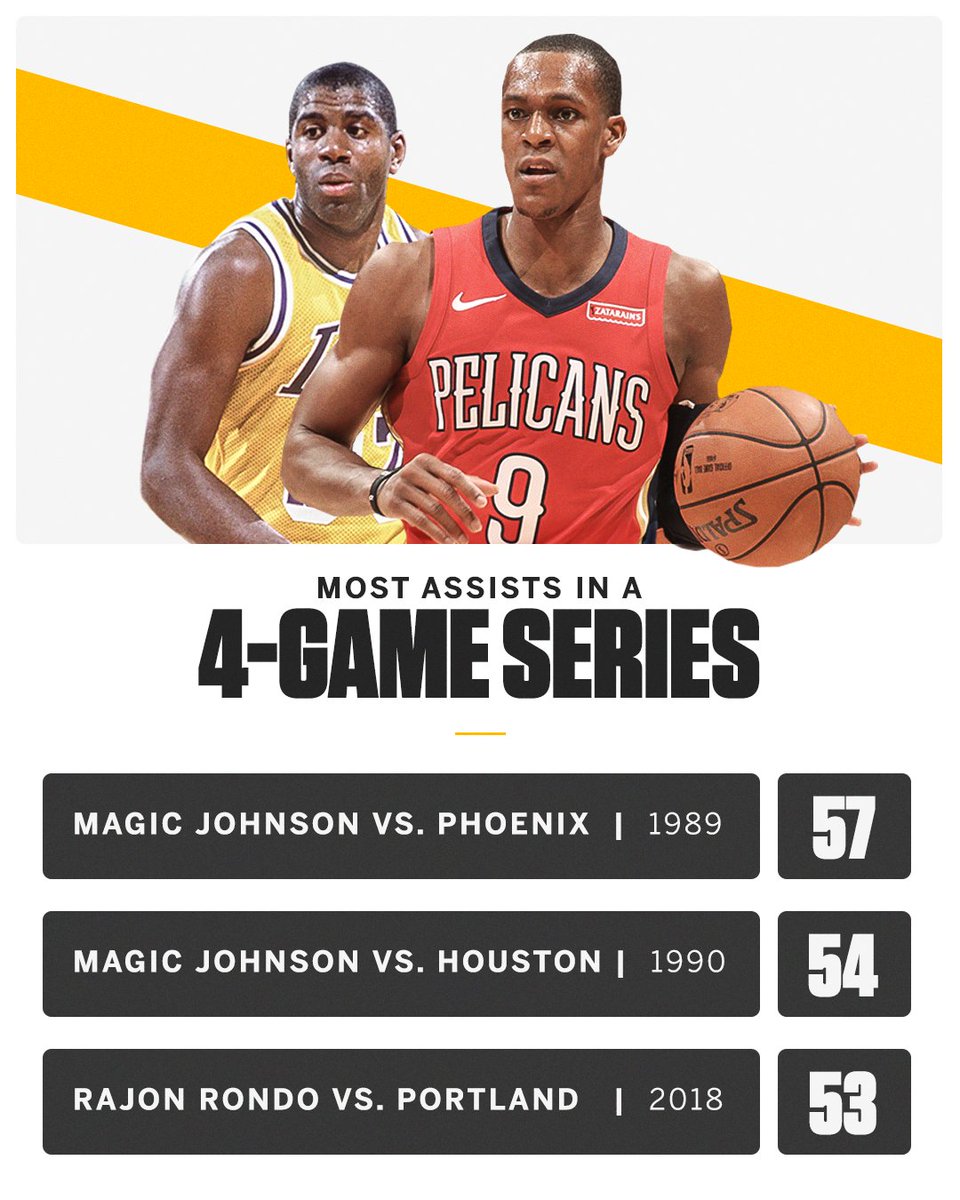The image features two basketball players from different eras and teams, captured in an action shot. In the forefront, a player from the New Orleans Pelicans, identified as Rajon Rondo, is dribbling the ball. Trailing behind him is the legendary Magic Johnson, wearing a yellow Los Angeles Lakers jersey, indicative of his playing days in his youth.

The graphic highlights the achievement of "Most Assists in a Four-Game Series," presenting data in black boxes. Magic Johnson's record is showcased with 57 assists against Phoenix in 1989 and 54 assists against Houston in 1990. Rajon Rondo's performance is also recognized with 53 assists against Portland in 2018. Diagonal yellow stripes accentuate the dynamic nature of the two players, against a minimalist white background that lacks additional text or headers beyond the main statistic.